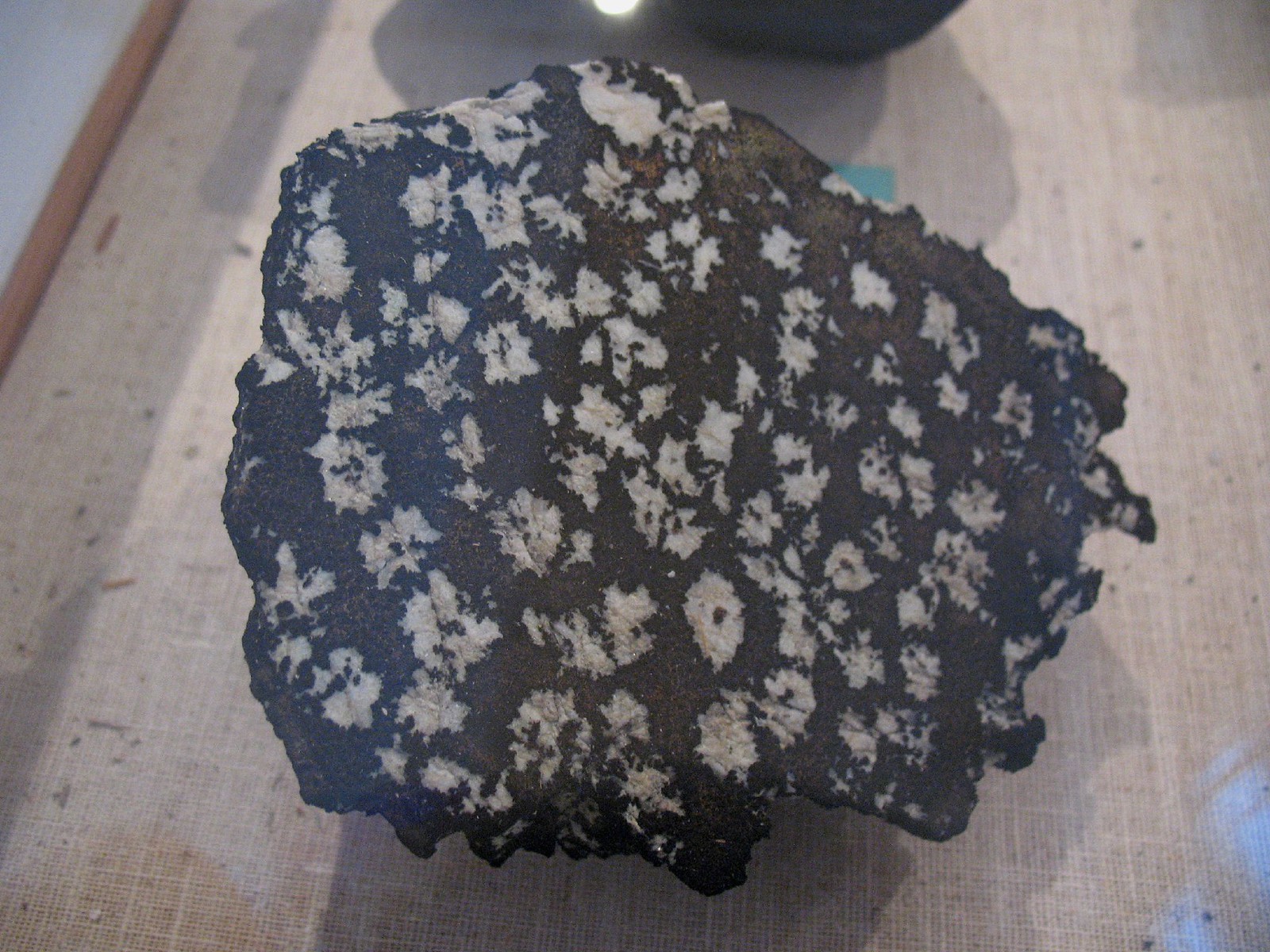The image is an up-close photograph of a rock resting on a tan-colored canvas with a brown wooden edge. The rock itself reveals a smooth face on one side and jagged edges, suggesting it may have been cut to expose its interior. The rock's surface is a dark, mossy green with brown tones, adorned with various random spots of gray or white that feature brown stripes running through these lighter areas. Reflective and glossy, the rock catches and refracts light, creating subtle reflections and highlights. Notably, there are white speckled dots across its coarse and textured edges, adding to its rugged appearance. The canvas it rests on is beige, and a light source from above casts shadows, including a shadow resembling the number one to the left. In the bottom right-hand corner, there is a faint light blue reflection, possibly from another nearby rock or object not fully in view.